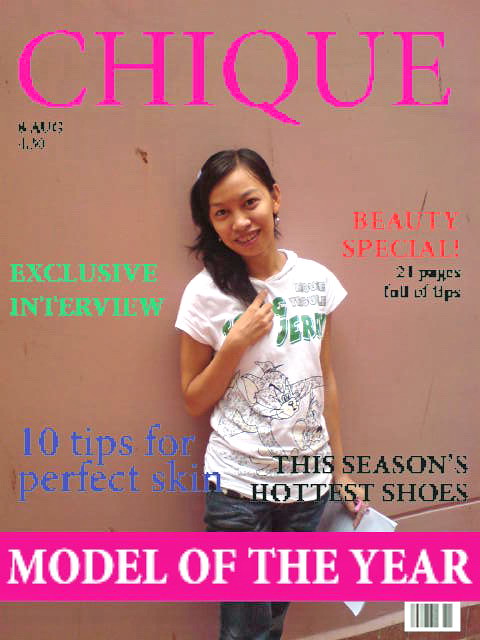The magazine cover features the title "Chic" in large pink letters across the top. Centrally placed is an image of a young woman standing against a pastel-tan or mauve-colored wall. She has long black hair cascading over her right shoulder and wears a white t-shirt with green text that reads "Tom and Jerry," accompanied by drawings of the cartoon characters below. Dressed in blue jeans, she poses with her right hand near the bottom of her hair and her left hand holding some paper at her side. The cover is full of various text elements: to her left in green print it says "Exclusive Interview"; to her right in red print it says "Beauty Special," with "21 Pages Full of Tips" in black underneath; to the left of her waist in blue text are "Ten Tips for Perfect Skin"; and spanning her waist and moving right, in black text, is "This Season's Hottest Shoes." A hot-pink band at the bottom says "Model of the Year" in white capital letters, with a barcode located in the lower right-hand corner.